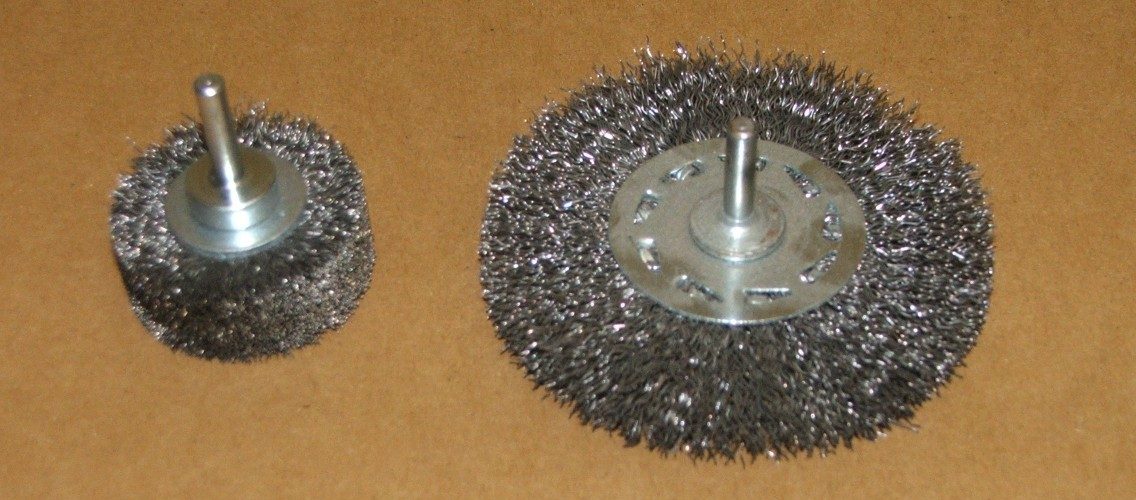The image features a brown background and showcases two silver metallic objects with circular shapes. The larger circular object displays intricate cutouts, resembling patterns stamped out of the metal. The objects glisten under a light source, enhancing their shiny appearance. Dark silver threads spread out from the larger circular object, giving the impression of silver fuzz or a filamentous material. This fuzz resembles the texture of a scouring pad used for dishwashing, with flatter fuzz around the larger circle and thicker fuzz encircling the smaller circle positioned to the left.